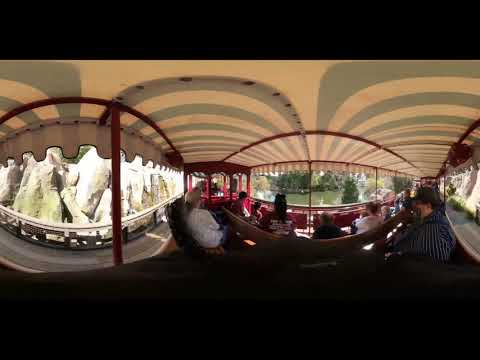This image presents a distorted, panoramic view captured with a 360-degree camera, causing the scene to warp into rounded shapes. It appears to depict an open-sided, trolley-like vehicle with burgundy metal framing and wooden brown seats. The vehicle features an overhead tarp, with alternating cream white and sage green stripes. Passengers are seated, seemingly focused in the same direction, indicating motion or a shared activity. The setting includes a wooden bridge on the left-hand side, a rocky wall, and a green body of water surrounded by trees. Large windows or open areas provide a clear view of the passing natural scenery, giving a sense of traversing through a lush, picturesque landscape.